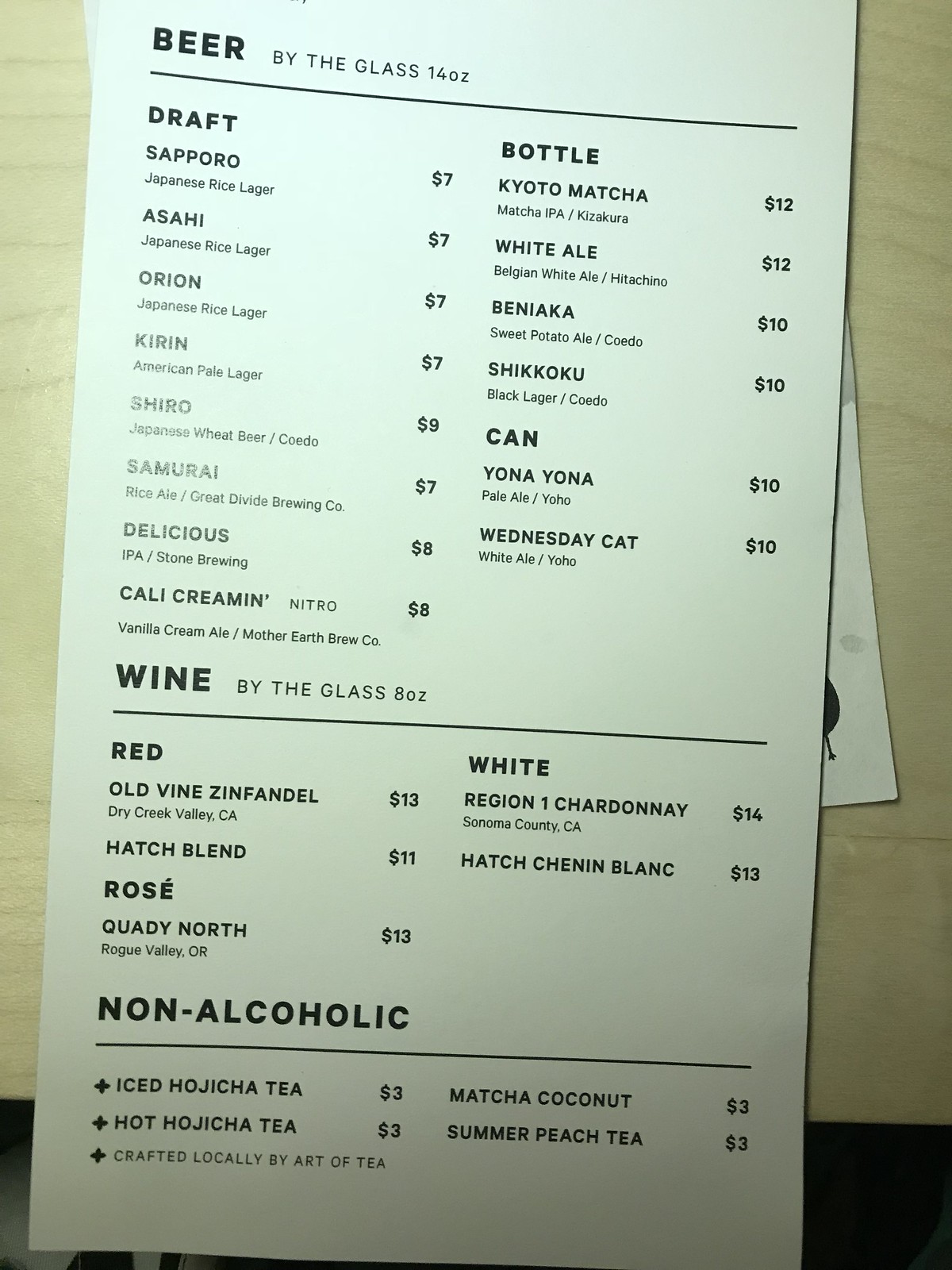**Detailed Menu Description on Brown Countertop**

Displayed prominently on a brown countertop is a detailed menu featuring an extensive selection of beverages. The top left section of the menu showcases the beer offerings in bold black lettering titled "Beer by the Glass, 14 ounces." The list includes:

- **Jap Sapporo** - Japanese rice lager, $7
- **Asahi** - Japanese rice lager, $7
- **Orion** - Japanese rice lager, $7
- **Kirin** - American rice lager, $7
- **Jiro** - Japanese wheat beer, $9
- **Tamarai** - rice ale, $7
- **Delicious** - Japanese, $8
- **Kelly Creamy Nitro** - Vanilla Cream Ale, $8

Bottled beer options are detailed next:

- **Kyoto Matcha** - Matcha IPA, Kizakura, $12
- **White Ale** - Belgian White Ale, $10
- **Black Lager**, $10

Canned beer selections include:

- **Yona Yona Pale Ale**, $10
- **Wednesday Cat** - White Ale, $10

The menu also features a section for wine by the glass (8 ounces) with the following varieties:

- **Red Wine**:
  - **Old Vines in Vandell** - Dry Creek Valley, California, $13
  - **Hatchbine**, $11
- **Rosé**:
  - **Quaddie North** - Rogue Valley, Oregon, $13
- **White Wine**:
  - **Region One Chardonnay** - Sonoma County, California, $14
  - **Hatch Chin and Blanc**, $13

A selection of non-alcoholic beverages is listed at the bottom, offering:

- **Iced Hojicha Tea**, $3
- **Hot Hojicha Tea**, $3
- **Matcha Coconut**, $3
- **Smoked Peach Tea**, $3

These non-alcoholic options are crafted locally by Arditea. The bottom of the menu appears to be slightly shadowed, adding a touch of depth to the display.